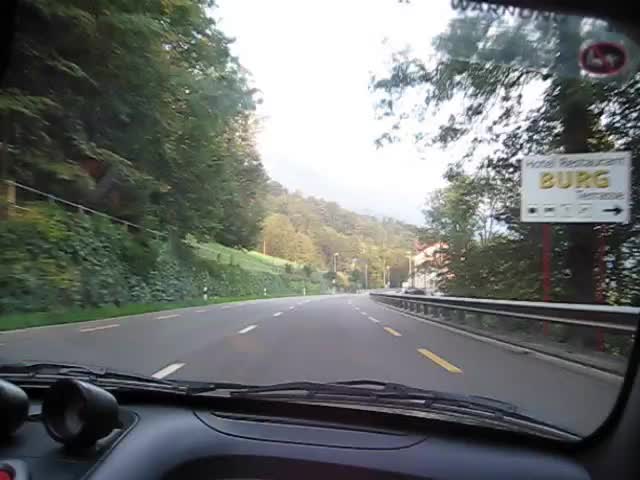The image captures a view from the passenger side of a vehicle's dashboard, with the photograph taken from the right-hand side. Prominently featured is a sign for a hotel and restaurant, mounted on a utility pole, with an arrow pointing to the right. The sign and most of the surroundings are blurred. In the background, you can see vegetation and trees lining both sides of the road, suggesting a rural setting. On the right, there's a building partially visible amongst the trees. The road ahead is empty, stretching out into the distance under an open daytime sky, enhancing the feeling of a serene, untraveled highway.